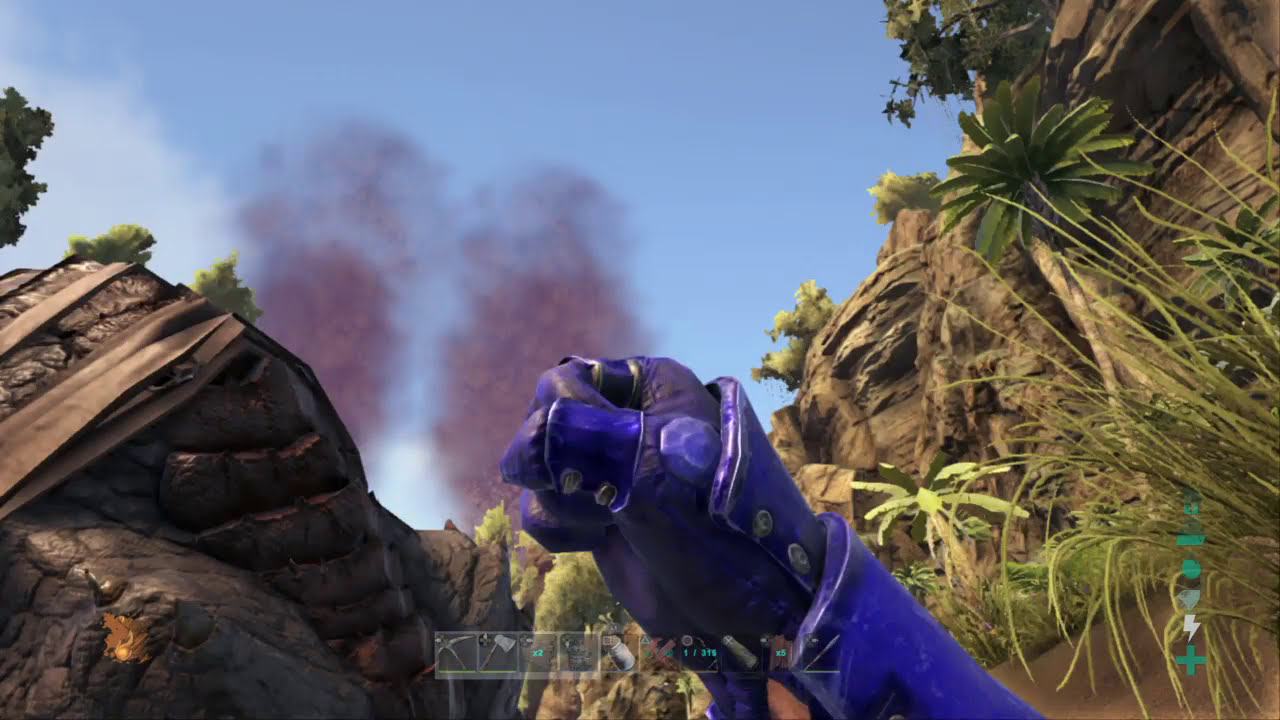This image is a screenshot from a video game depicting a dramatic nature scene. At the center of the image is a prominently raised fist, clad in a royal purple or blue armored glove, complete with detailed buttons and a gauntlet. The arm wearing the glove is slightly visible, and the hand is in a clenched position, commanding attention against the backdrop. The background features a vibrant blue sky with columns of purple-gray, dark smoke rising in the distance. The scene appears to be set within a canyon, bordered by tall cliffs adorned with tropical foliage, including ferns or palm trees, and a substantial boulder on one side. The boulder appears to have a plank or some unknown object laying across it. Surrounding the fist and cliffs, the landscape is rich with green vegetation, trees, and shrubs, juxtaposed against the earthy tones of the rocky formations. Additionally, the image contains some cryptic symbols in the lower part and on the right, reinforcing the video game setting.